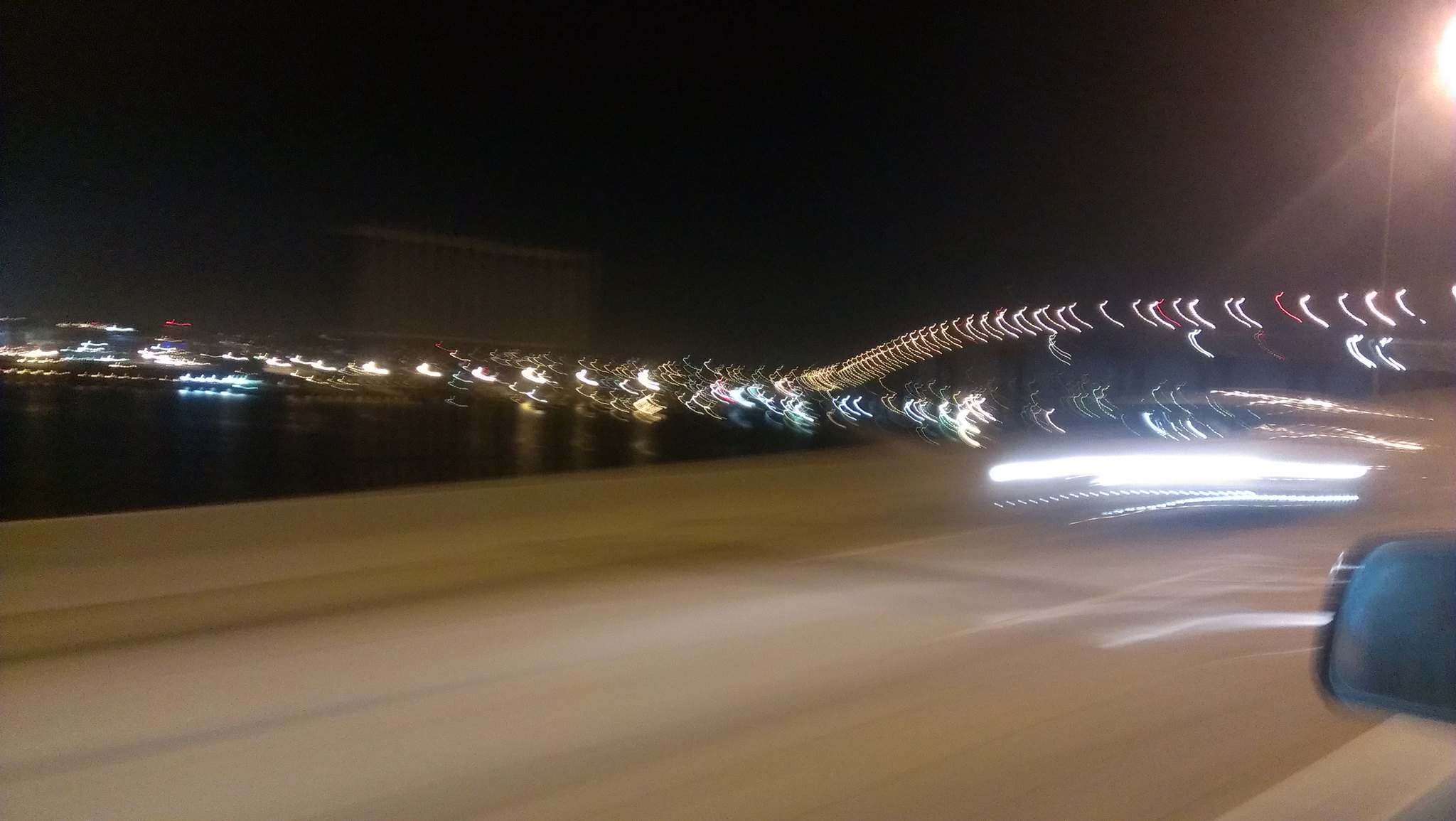This nighttime photograph, taken from the side window of a moving car, captures a dynamic urban scene filled with intricate light patterns. The road, an expansive light gray surface, is dimly illuminated by overhead street lamps. To the left, a concrete divider wall blurs into the motion. A string of J-shaped lights stretches along the scene, forming a repetitive pattern that continues into the distance. On the left side, a bustling cityscape reveals buildings outlined with glowing lights. These structures are reflected in the long lines of car lights, streaming left and right toward an intersection. The sky above is a deep, uninterrupted black, highlighting the vibrant urban hues below—white, yellow, blue, and hints of pink. Near the bottom right corner, the blue hue of the side mirror identifies the car’s presence, while another blurred, bright light in the center right indicates another vehicle. Across the riverbank, anchored beyond the road, stands a large rectangular building that towers over the scene, its grey façade barely visible in the ambient light. The photograph encapsulates the spirited energy of a city night, viewed fleetingly through the window of a speeding car.